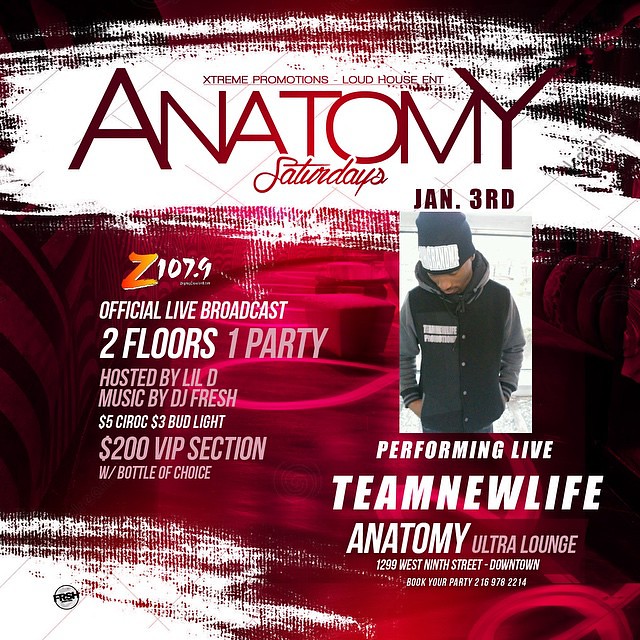This is an advertisement for "Anatomy Saturdays," a house music event hosted by Loud House Entertainment and Extreme Promotions. The prominent visual theme features a vibrant red background with an overlay of white and black graffiti-like elements. At the top, in small red font, the text reads "Extreme Promotions Loud House Ent." Below it, in larger red font, "Anatomy" is displayed, followed by "Saturdays" in a red cursive style. To the right is the event date, "Jan 3rd," in dark red font.

The image includes key promotional details such as "Z107.9" in a gradient red to orange font, followed by "Official Live Broadcast" in white. The event boasts "Two Floors, One Party," and it's hosted by Lil D with music by DJ Fresh. Drink specials include $5 Ciroc and $3 Bud Light, while there's a $200 VIP section that includes a bottle of choice.

A vertically cropped photograph to the right features an African-American man looking downwards with his hands in his jacket pockets. He is wearing a black beanie with a white design and a button-up jacket in black and dark gray. This indicates "Performing Live, Team New Life."

Additional details include the venue, "Anatomy Ultra Lounge, 1299 West 9th Street, Downtown," and a call to action to "Book Your Party" with the contact number 216-978-2214. The background is dominated by dark red with box-like designs at the center, adding to the event's high-energy promotional aesthetic.